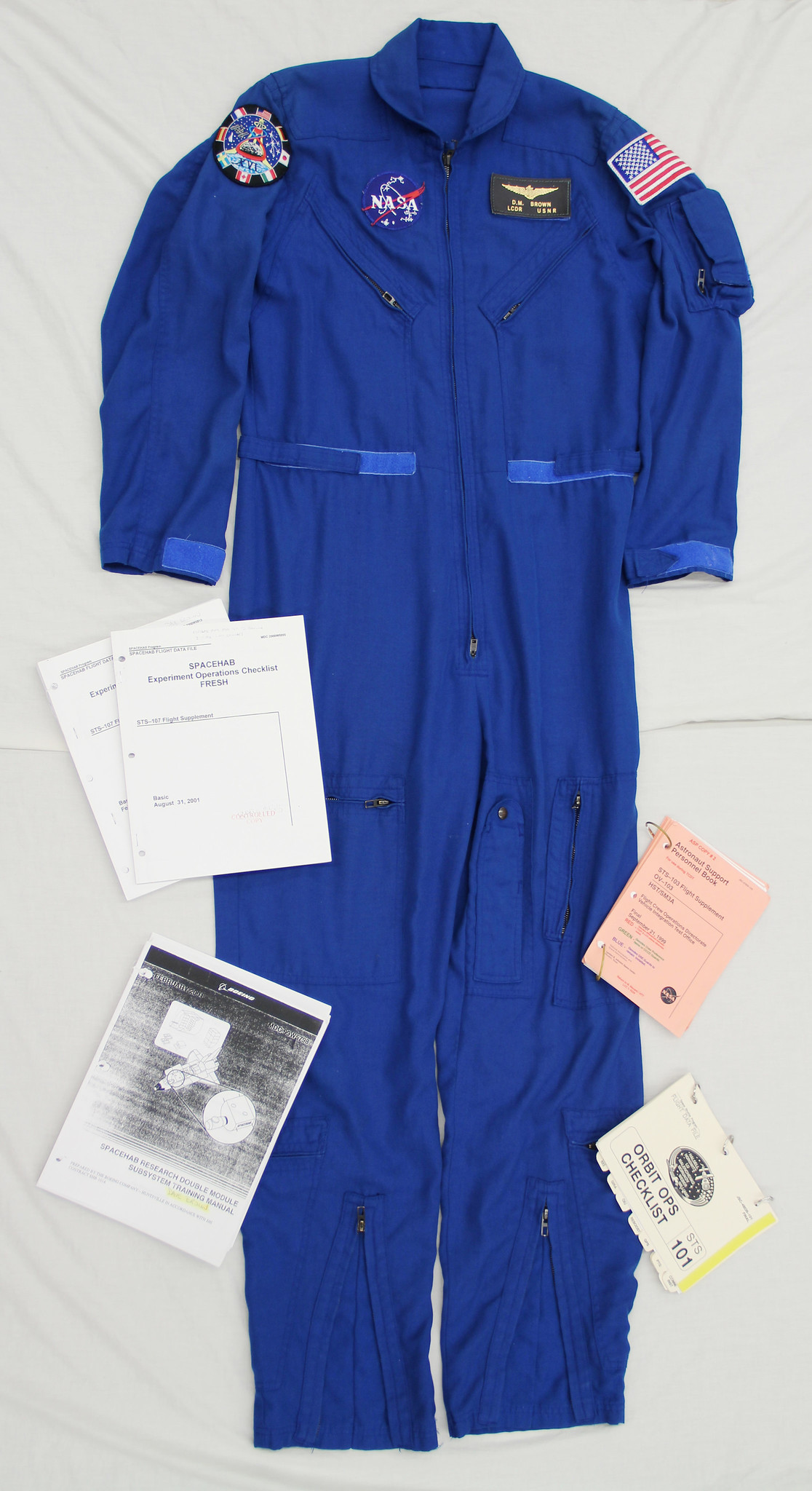This detailed color photograph showcases a NASA astronaut's dark royal blue flight suit intricately laid out on what appears to be a white cloth background. The one-piece jumpsuit features a variety of patches and zippers, highlighting its functional and symbolic design. On the left shoulder, there is a prominent American flag patch. The right shoulder also displays another American flag patch, positioned just above a shoulder pocket with a black zipper. The suit's chest is adorned with several significant emblems: the left chest area has a NASA logo, and adjacent to it is a flag pin emblem for the US Air Force. 

On the left side of the suit, a patch with a space shuttle design can be seen, embellished with various flags including those of Japan, Italy, Canada, Spain, America, and Germany. Two diagonal black zippers cross the center of the torso, adding to the suit's intricate detail. The suit extends into long royal blue pants. Alongside the suit, there are pieces of paraphernalia: a white item labeled "space HAB," another displaying a space shuttle scan, a pink booklet, and a white booklet titled "orbit OPS checklist 101" in black ink. Additionally, there are other sheets of paper, one notably featuring a mix of gray and black images and text, providing context to the suit's elaborate setup. This photograph not only captures the essence of a NASA flight suit but also the meticulous preparation involved in space missions.